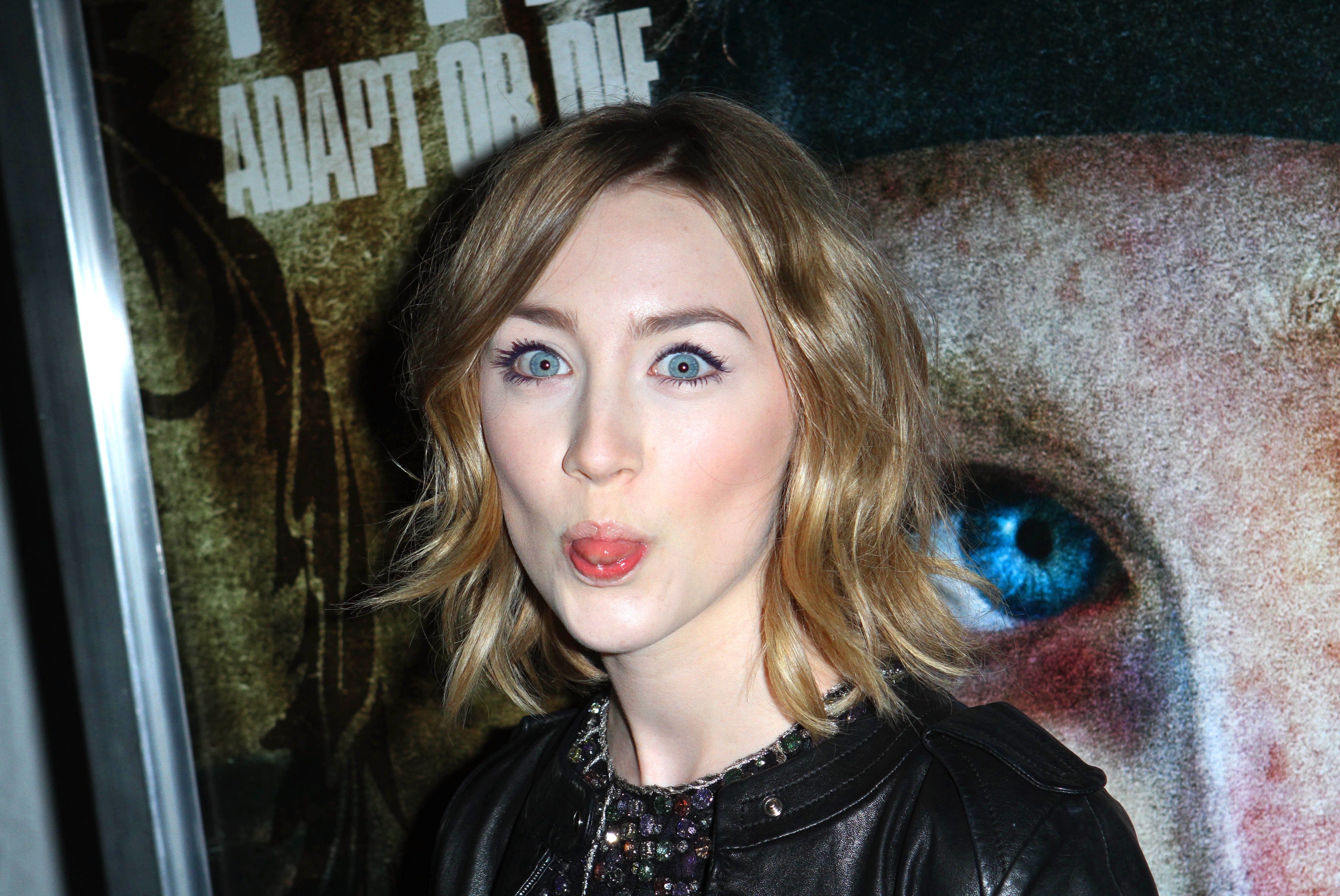In this photograph, the Irish actress Saoirse Ronan stands in the center, striking a whimsical pose by sucking in her cheeks and sticking out her tongue. She wears a black leather jacket over a bejeweled or intricately patterned dark dress, which shimmers under the camera flash. Her shoulder-length, wavy blonde hair slightly obscures her ears, which are hidden from view. Her light, icy blue eyes are accentuated with eyeliner, and her cheeks, lightly brushed with blush, give her a vibrant yet playful appearance. The background features a promotional poster for the movie "Hanna," prominently displaying the phrase "Adapt or die" in white text. The poster also includes a close-up of a face with a striking blue eye, particularly noticeable behind Ronan on her right. The overall lighting suggests an event setting, adding to the lively and cheerful vibe of the image.